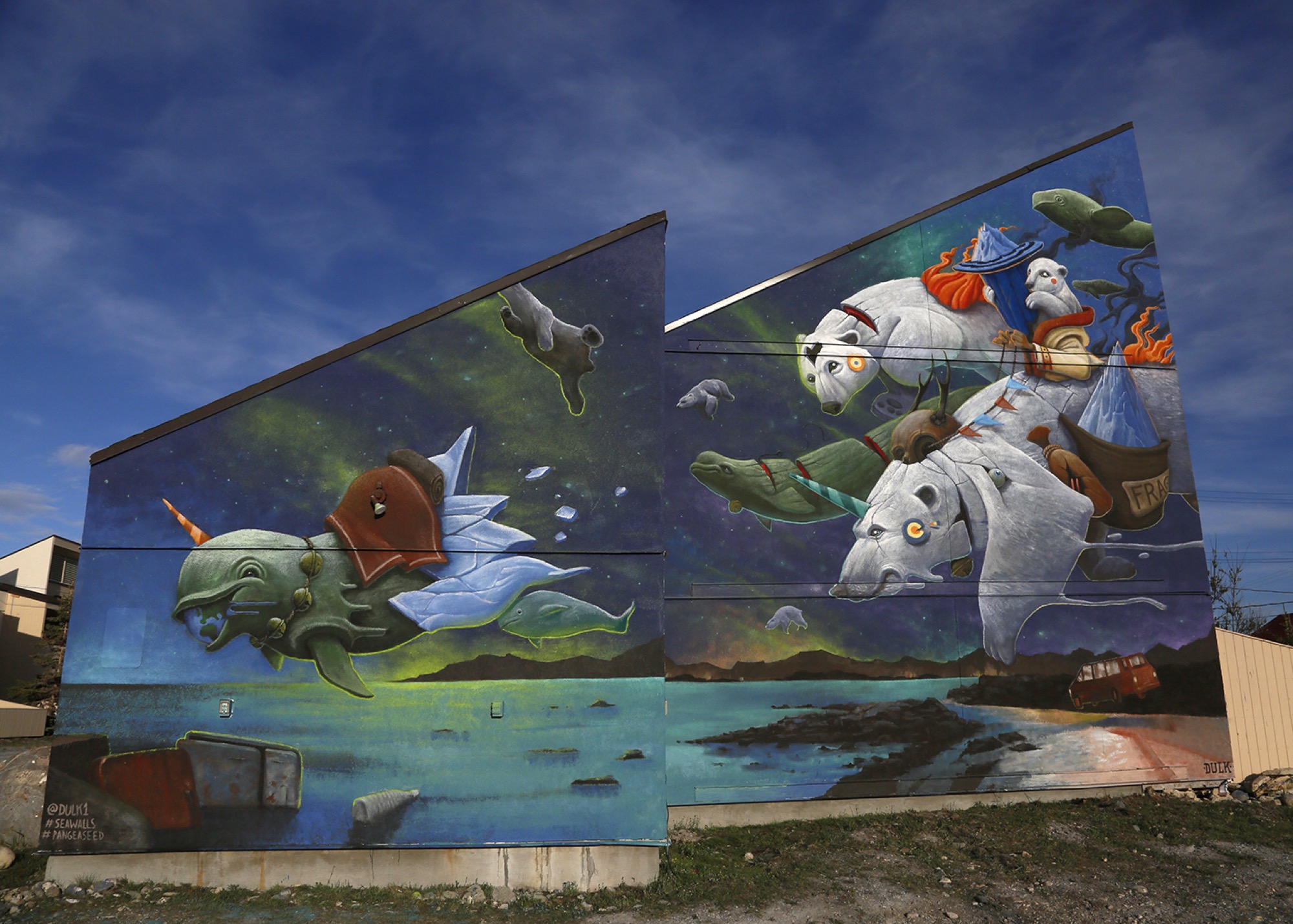Captured against a bright blue sky dotted with light clouds, the image features an intricate and colorful mural encompassing multiple panels of a slanted, partially obscured wall, resembling a billboard or part of a building. The artwork, rich in detail, blends computer-generated and hand-drawn graphics to depict a surreal seascape populated by fantastical animals. 

In the foreground, a dolphin with a unicorn-like horn delicately balances the Earth in its mouth, adorned with a bald necklace and an icy blanket trailing off its tail. Nearby, a horned bear carries a sack with ice spilling out, while another large horned bear appears with strange companions—a leopard encased in a coat with arms and a red pillow or possible flame in its background. The sea beneath them is littered with trash, including bottles, signifying pollution.

The mural transitions seamlessly into a landscape of imaginative creatures: a green whale, flying bears, and other animals, all set against a night sky filled with stars. This fantasy art is contrasted sharply with the real-world setting around it, an urban neighborhood or industrial park, and even a van can be seen near the edge of the sea in the foreground.

At the bottom left of the mural are hashtag tags, possibly reading "#Cwalls" and "#ManageC." The entire scene blurs the lines between reality and imagination, aiming to draw viewers into a whimsical world where the depicted water and land appear almost real—a fantastical window to another realm juxtaposed against the mundane backdrop of the surrounding area.